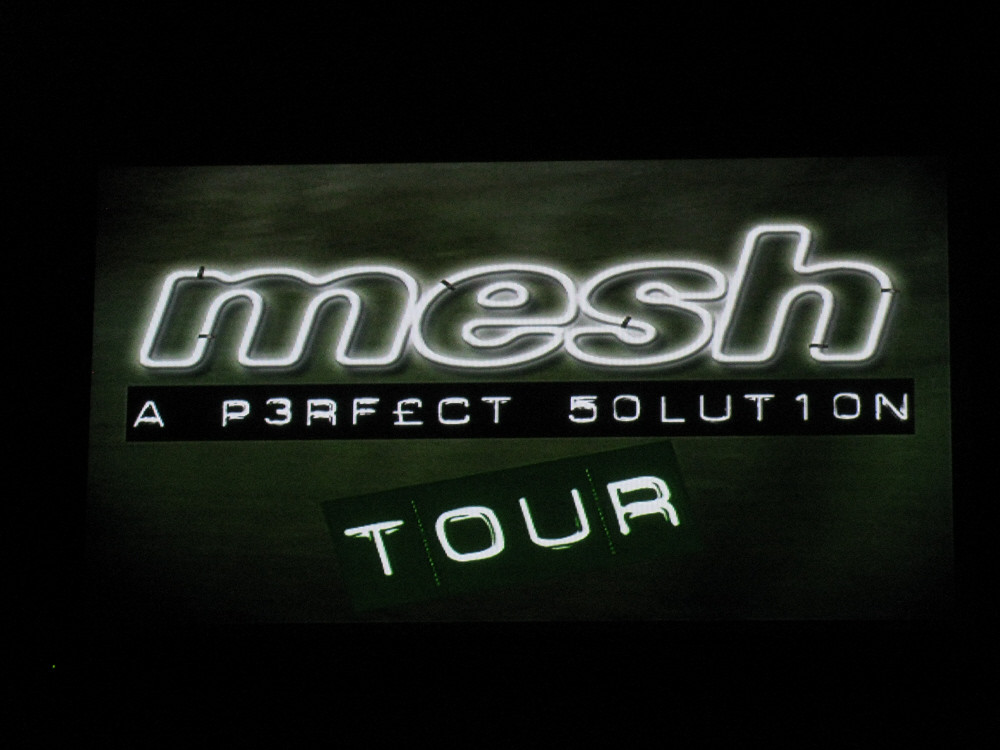The image showcases a striking advertisement set against a flat black background. Centered in this dark backdrop is the word "mesh" rendered in large, lowercase white letters with a captivating neon glow effect, giving it a striking, illuminated appearance. Directly beneath “mesh,” in a smaller, unique and creatively spelled text, it says "P3rf€ct 5olution" in white, resembling label maker output with a playful use of special characters to form the words. Below that, in matching white text and all capital letters, is the word "TOUR" angled slightly upwards, adding a dynamic touch. The overall design contrasts the sleek, neon-like digital art of the word "mesh" against the minimalist black background, with the subsequent text elements providing an intriguing and visually appealing blend of styles.